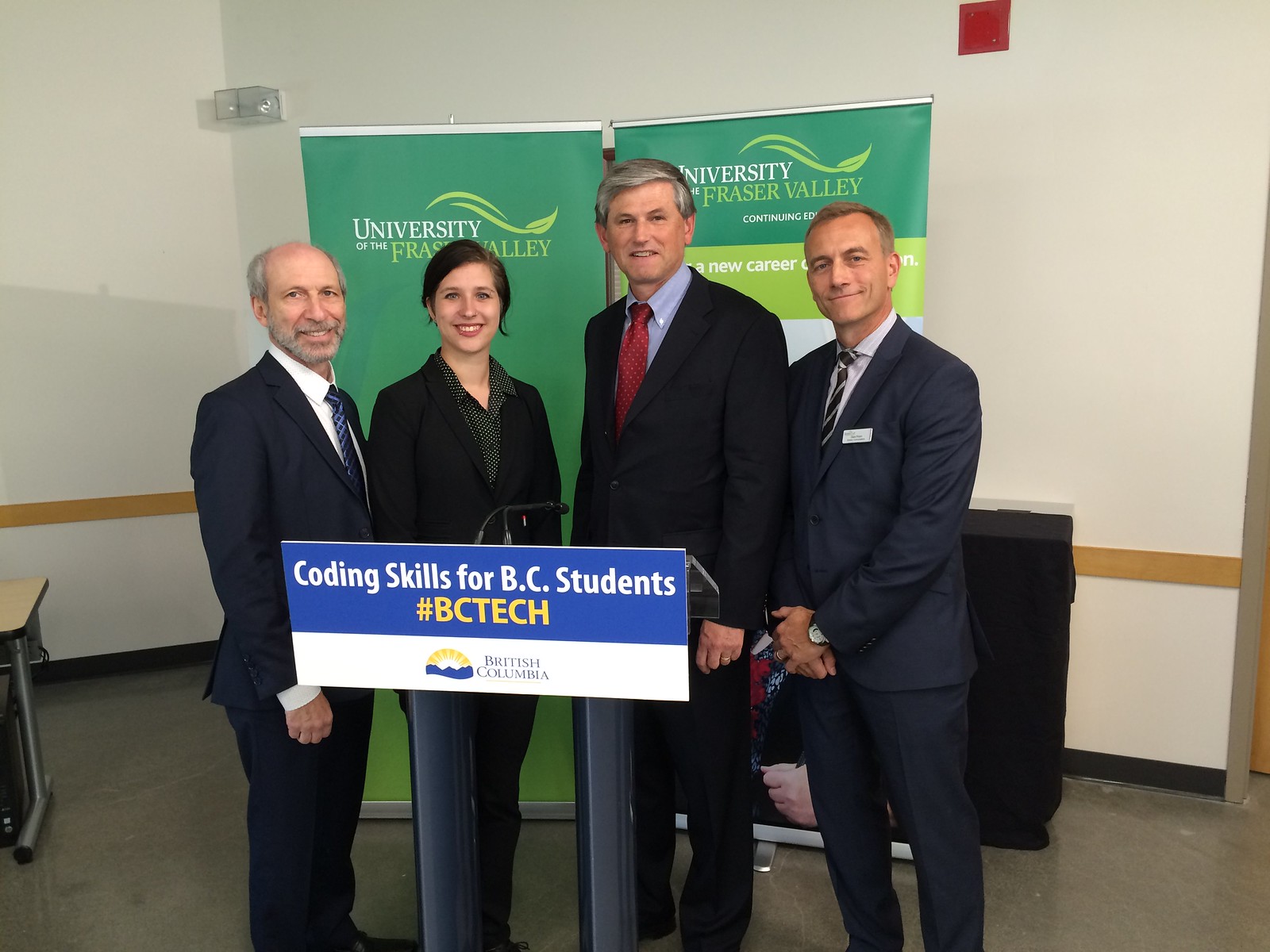The photograph, taken indoors, features four white adults posing at the center. From left to right, the first individual is an older man, nearly bald with a little gray hair on the sides, dressed in a dark blue suit with a white shirt and blue tie. Next to him is a woman with dark hair pulled back, wearing a black suit over a dark gray shirt. She is followed by a man with thick gray hair and a smile, dressed in a dark suit that is nearly black or dark blue, a blue shirt, and a red tie. The last person is a man with short hair, donning a dark blue suit with a white shirt and a black and white tie. They are all in business attire.

They stand in front of a podium with a microphone, adorned with a banner that reads "Coding Skills for BC Students, #BCTech." Behind them is a backdrop featuring the green text "University of the Fraser Valley." The setting suggests the photograph was taken in a university classroom or similar academic environment, evidenced by the design of the off-white wall with a black baseboard and wooden molding at waist level, likely to prevent scuffs.